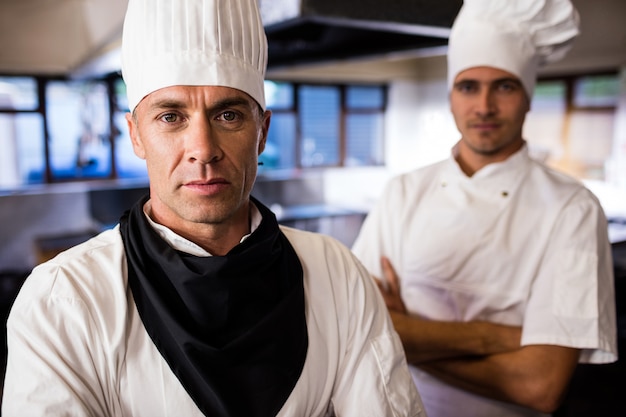The photograph captures two chefs in an indoor, kitchen setting. Both men are donning white chef uniforms and white chef hats. The chef on the left, who is the primary focal point, stands in sharp focus with his arms crossed, looking directly at the camera with serious brown eyes. He has a hint of beard stubble and is distinguished by a black neckerchief tied around his neck. The chef on the right is slightly out of focus and also has his arms folded across his chest. The background, presumed to be part of the kitchen, is blurred but reveals windows, walls painted white, and a glimpse of a sink. Both chefs display a serious demeanor as they pose for the photograph.